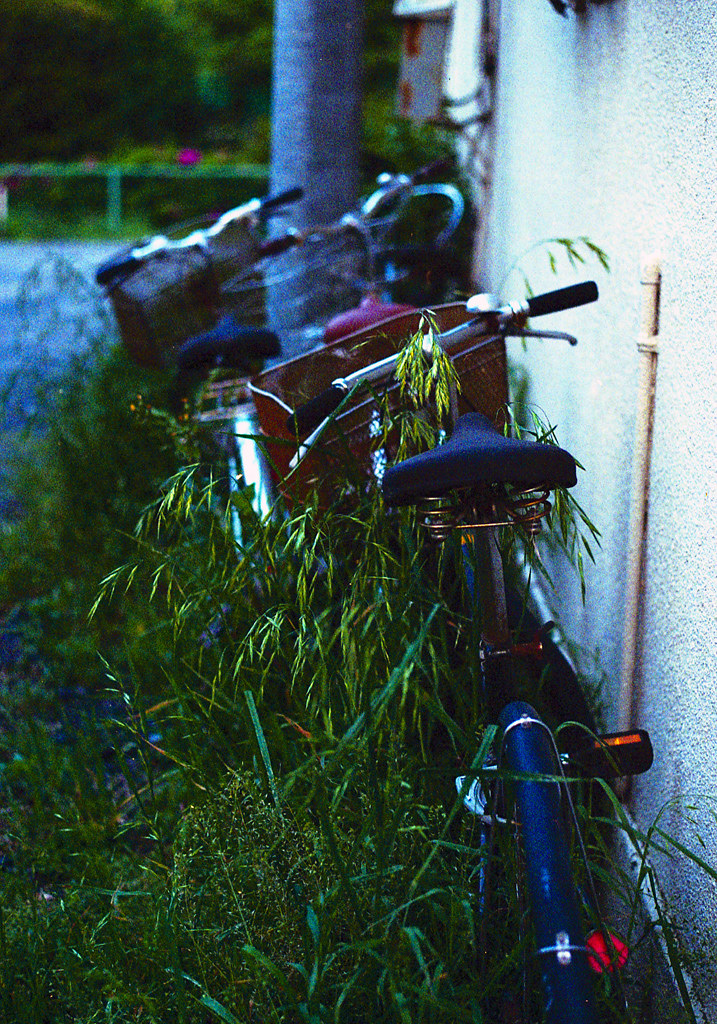The vivid color photograph captures an outdoor scene dominated by tall, wheat-like grasses and lush weeds enveloping a group of bicycles. The focal point is a gritty red bicycle with a wide, cushioned seat with springs, leaning against a white stucco wall adorned with electrical conduit. Nearby, additional bicycles—including a blue one with a matching blue seat and a silver one with a black seat—can be seen partially obscured by the overgrown vegetation. In the background, a large tree trunk rises beside the wall, and a fence adorned with blooming pink flowers and framed by trees stretches across the left side of the image. The saturated hues and rich details contrast with the slightly blurred focus, enhancing the rugged charm of the scene.